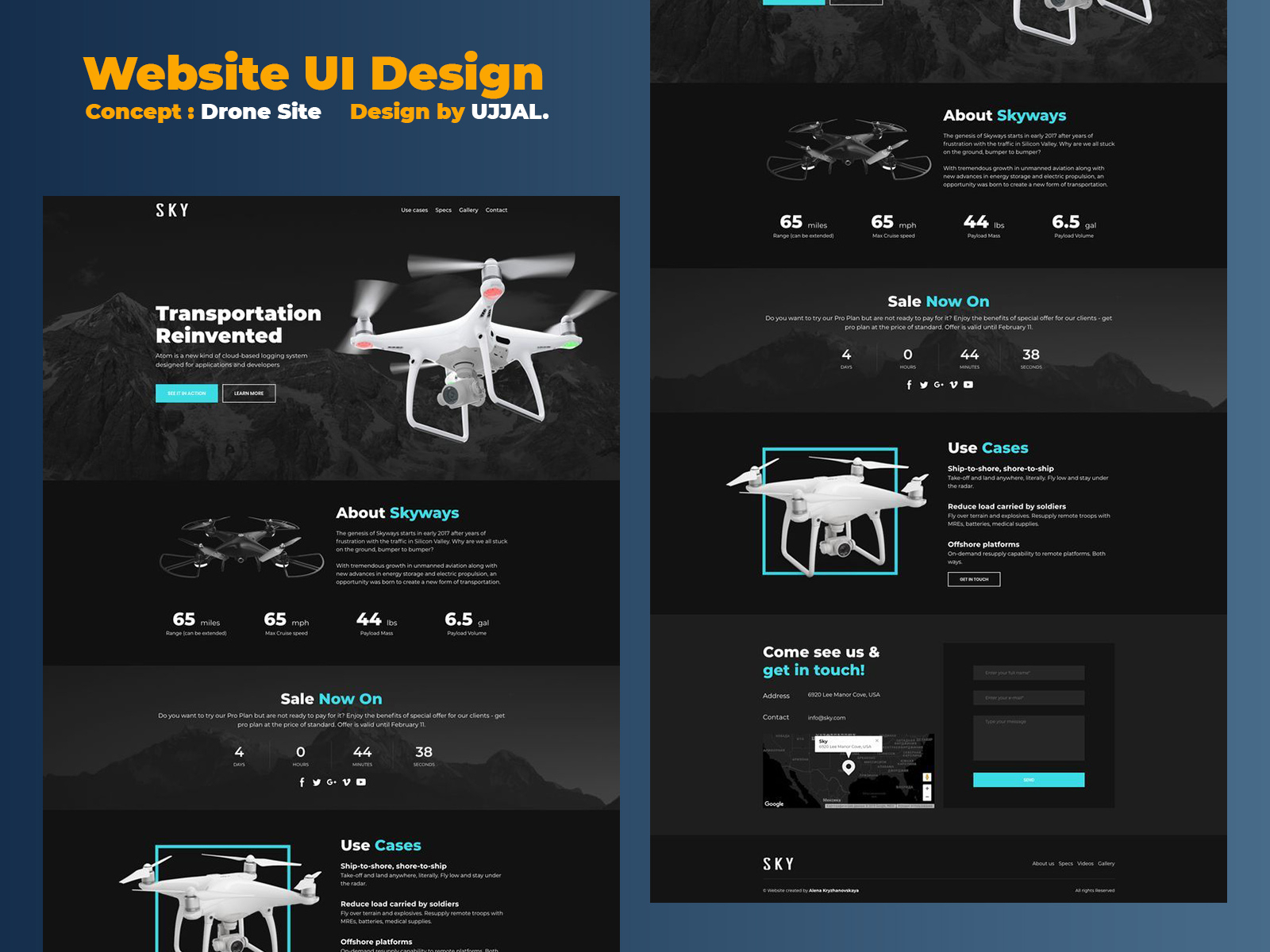This partial screenshot showcases a website UI design concept for a drone site, created by U33AL. The primary background is a deep navy blue. Central to the image are two side-by-side long rectangular graphics set against a nearly black backdrop. 

In the upper left corner, a piece of orange text reads, "Website UI Design Concept Drone Site Designed by U33AL."

The left graphic features an infographic with a prominent white personal drone, with motion-blurred blades in action. The infographic is sequentially arranged:
- The heading, "Transportation Reinvented."
- An image of the drone in flight.
- A section titled "About Skyways," followed by illegible text content.
- A call to action, "Sail Now On."
- The heading "Use Cases," paired with another image of the drone and additional unreadable text.

The right graphic mirrors the left one but displays the drone from an alternate angle.